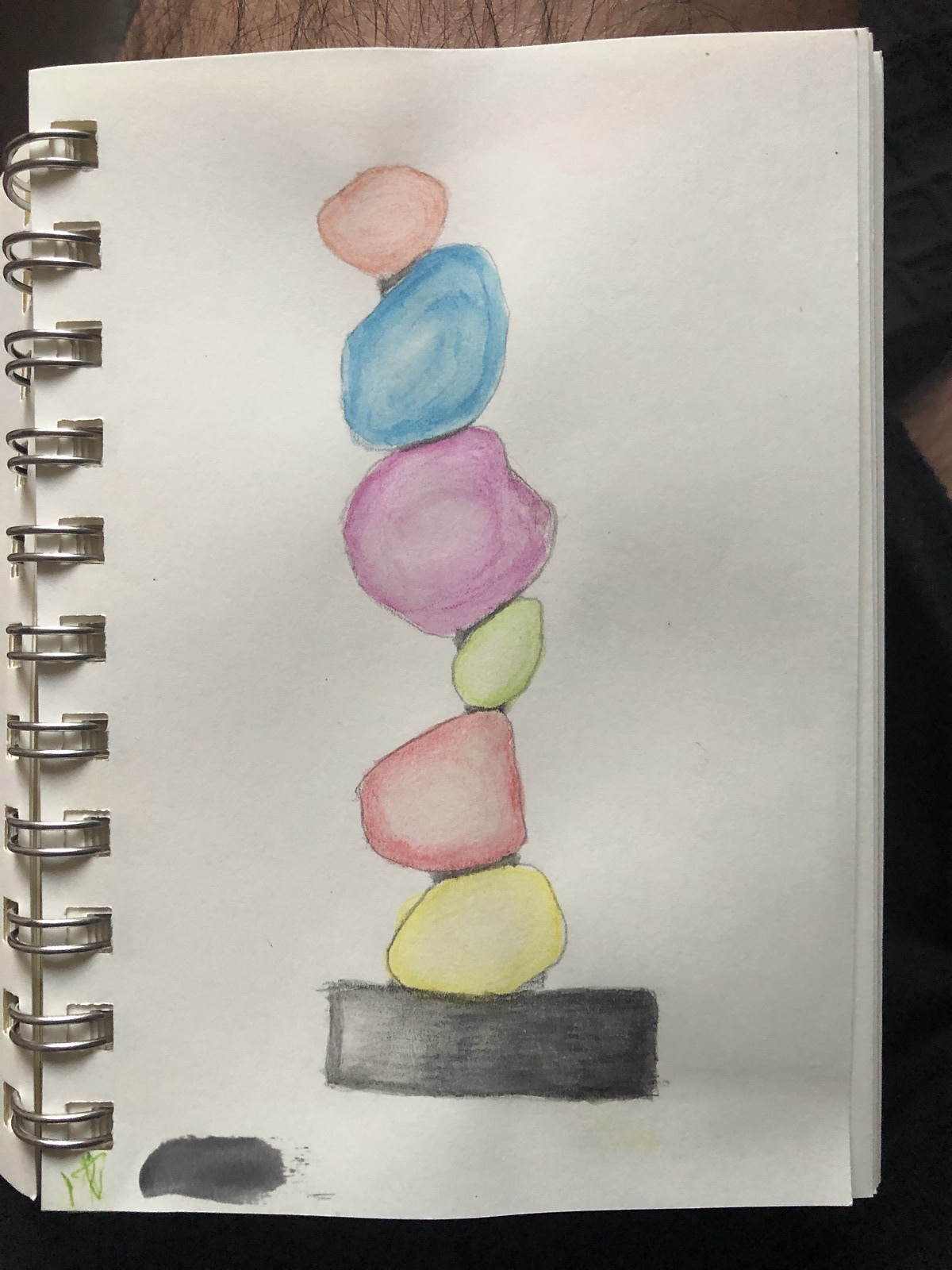A detailed descriptive caption for the image could be:

"Displayed is a watercolor painting on a white sheet of paper secured in a binder with a silver metal binding, visible through punctured holes along the side. The painting features a black rectangular base with six colorful stones precariously stacked on top. From bottom to top, the stones are painted in yellow, red, green, purple, blue, and orange. The vivid colors contrast sharply against the white paper, making the wobbly tower stand out. In the bottom left-hand corner of the sheet, there is a small swatch of black paint, likely used to test the color before applying it to the main artwork."